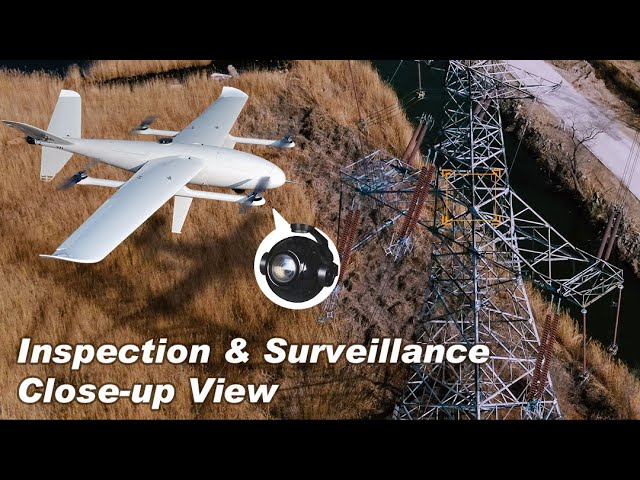This image, a composite of color illustration and photography, features a white propeller airplane, resembling a drone, flying over a dry, grassy field with rocky high ravines. The airplane, depicted in a screenshot-like frame, lacks windows or door openings and is equipped with a round, black camera mounted underneath its front section. This camera is highlighted in a close-up view within a white word bubble that includes an arrow pointing towards it. The camera, depicted with a glass front and side arms, suggests it has the capability to pivot. The plane also flies near large power towers situated on the upper right of the image. The overall scene has a landscape orientation, with the phrase "inspection and surveillance close-up view" written in italicized white text at the bottom left.